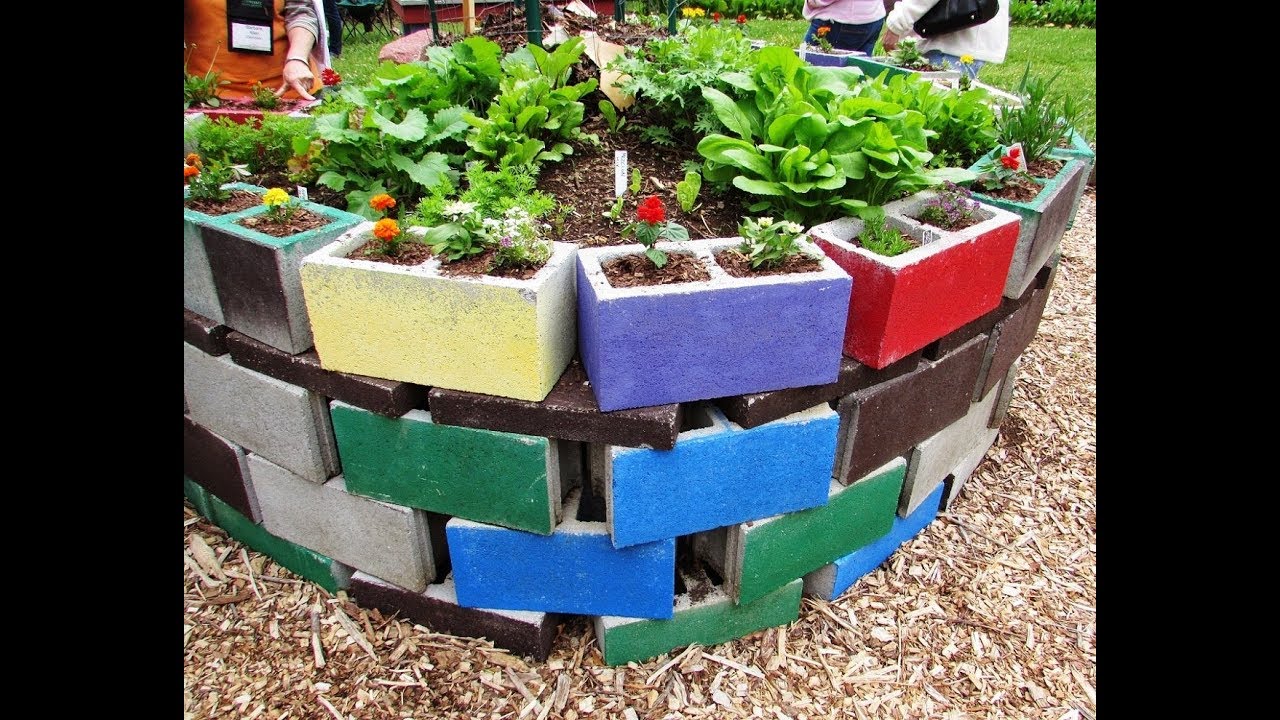This detailed photo captures a raised, circular garden bed ingeniously constructed using multicolored concrete blocks. The blocks, stacked atop one another, feature a variety of vibrant hues—light blue, green, yellow, and purple—that add a decorative edge to the planter. Each block's two square holes are creatively repurposed as mini planters, filled with brown dirt and blossoming flowers, including red, orange, and yellow blooms. The center of the circle houses a large garden bed filled with dark brown soil and lush, leafy vegetation. The garden area, possibly part of a community space or park, is set against a backdrop of concrete blocks and wood chips. In the rear of the photo, several people can be seen from the waist down—one woman in a pink shirt and jeans and another in a long-sleeve white shirt and jeans—adding a sense of scale and community engagement to this tranquil garden scene. The sky above is overcast, lending a cool, serene atmosphere to the setting.